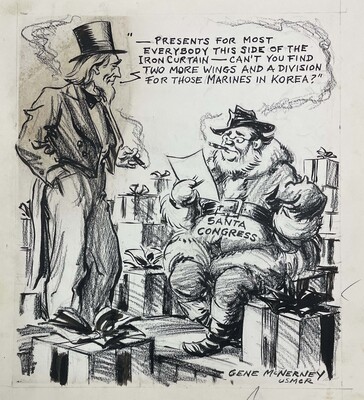This detailed black-and-white political cartoon, seemingly created with pencil or charcoal by artist Gene McHenry, showcases a critique from the Korean War era. The illustration features a portly man labeled "Santa Congress" seated and smoking a cigar, surrounded by elaborately wrapped gifts and boxes. Santa Congress is depicted scrutinizing a list, symbolizing governmental excess. Standing beside him, a figure resembling an older rendition of Uncle Sam—complete with long flowing hair, a beard, a top hat, and an old-fashioned coat and pants—holds a cigar and speaks to Santa Congress. Uncle Sam's speech bubble reads: "Presents for most everybody this side of the Iron Curtain. Can't you find two more wings and a division for the Marines in Korea?" This pointed message highlights the cartoon's critique of Congress's lavish spending while allegedly neglecting military needs.